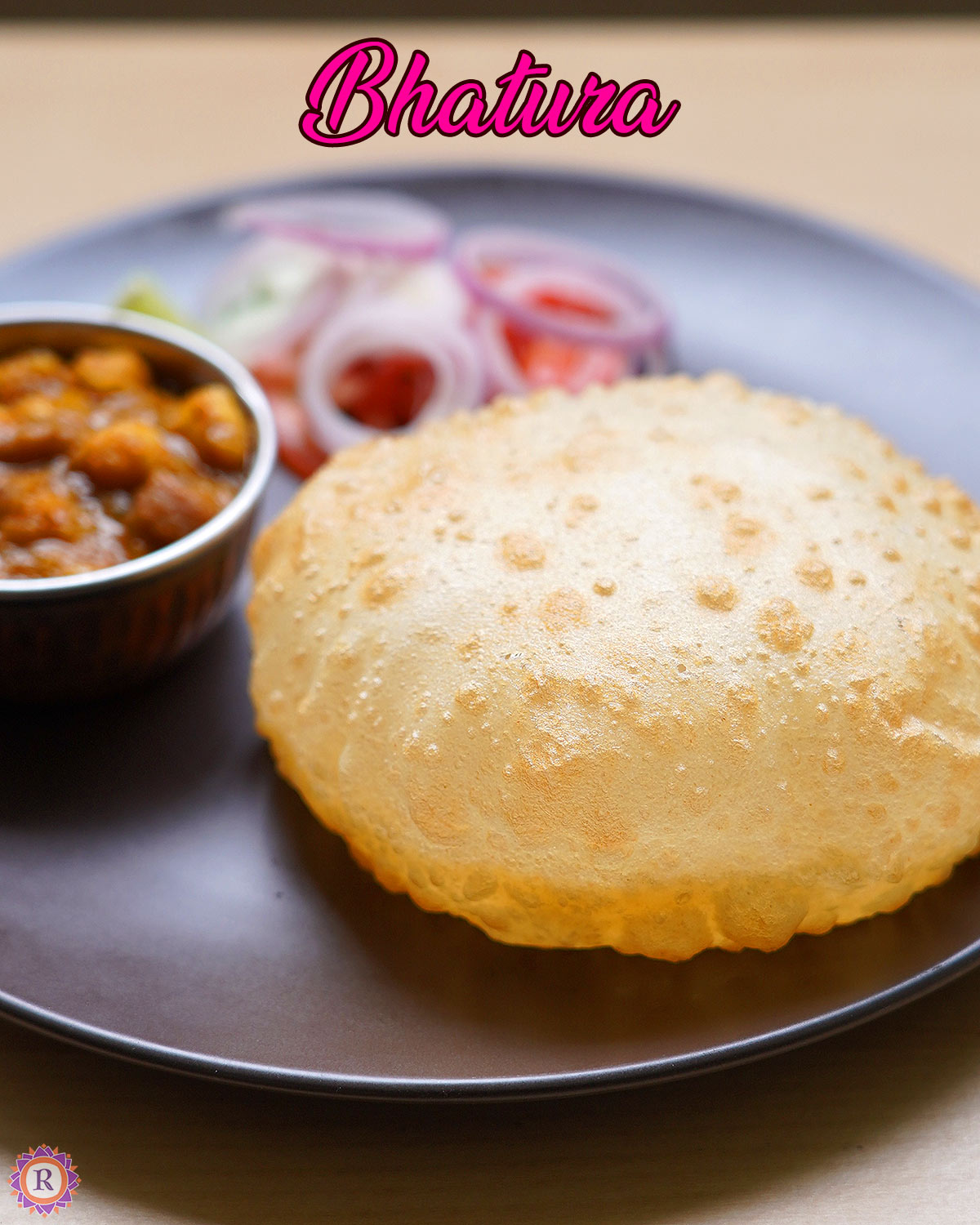This detailed color photograph captures a beautifully arranged plate of Indian food set against a blonde wood tabletop. In the top portion of the image, the word "Batura" is prominently displayed in pink script outlined in black. A dark-colored, possibly black or brown ceramic plate with a subtle white and black border at the edge serves as the base for the food.

On the lower right corner of the plate, there is a round, poofed-up piece of bread known as a puri, characterized by its light brown bubbly surface and slightly darker edges. Positioned centrally to the left of the puri is a small circular bowl containing a rich, lumpy orange curry with chickpeas. The upper part of the plate features a colorful salad of sliced raw onions and tomatoes, adding a fresh touch to the presentation.

In addition, the lower left corner of the photograph reveals a logo, encircled in white with a distinct purple 'R' and adorned with surrounding purple flower petals, further adding to the aesthetic appeal of the image.